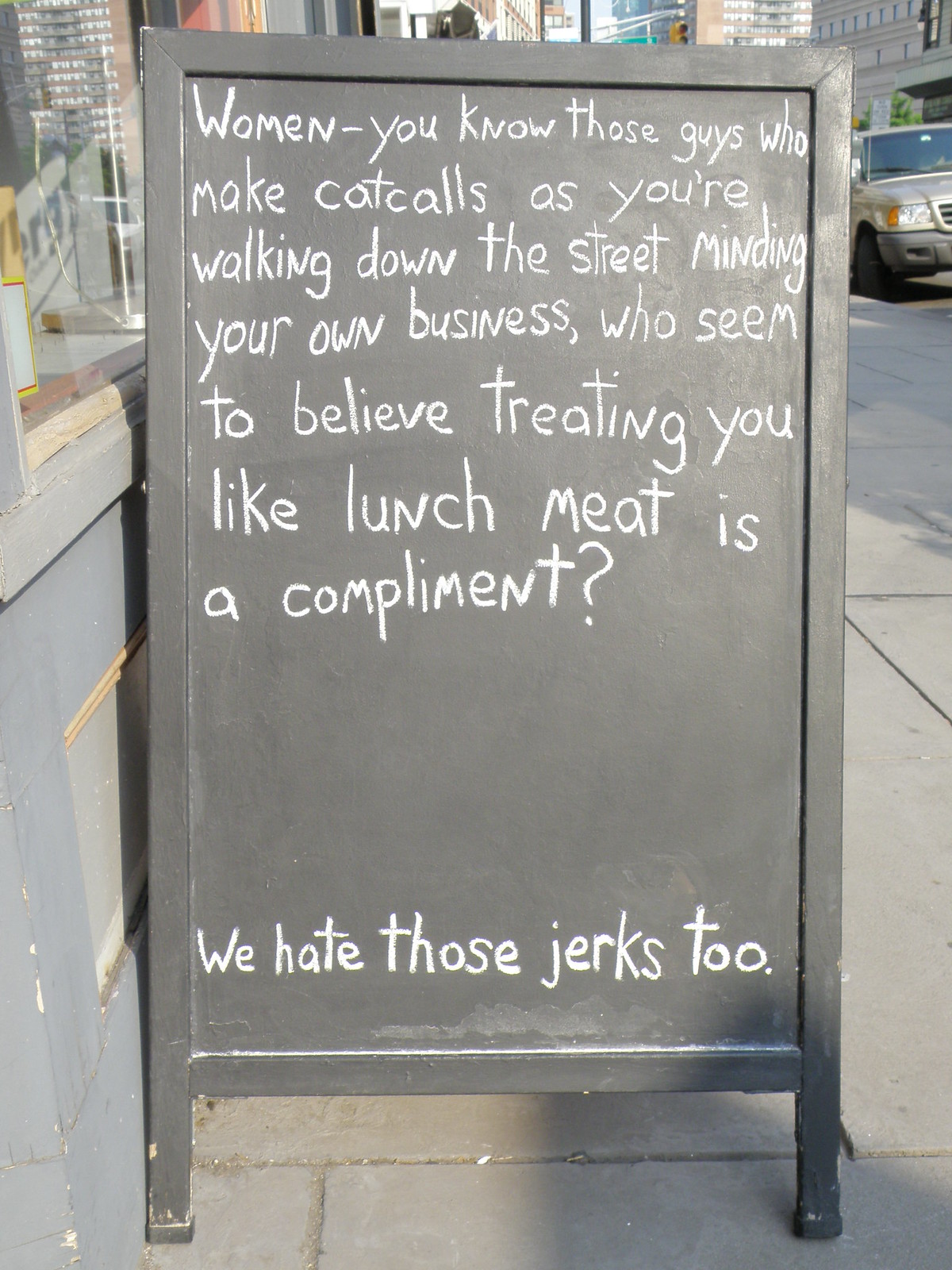The image features a black chalkboard sign placed against the wall of a store. The sign is written in white chalk and reads, "Women, you know those guys who make catcalls as you're walking down the street minding your own business, who seem to believe treating you like lunch meat is a compliment?" Underneath a blank space on the lower part of the sign, it adds, "We hate those jerks too." To the left of the sign, there is a building, while on the right side, a street scene unfolds. This includes several buildings in the background, a car, street signs, and a lamppost.